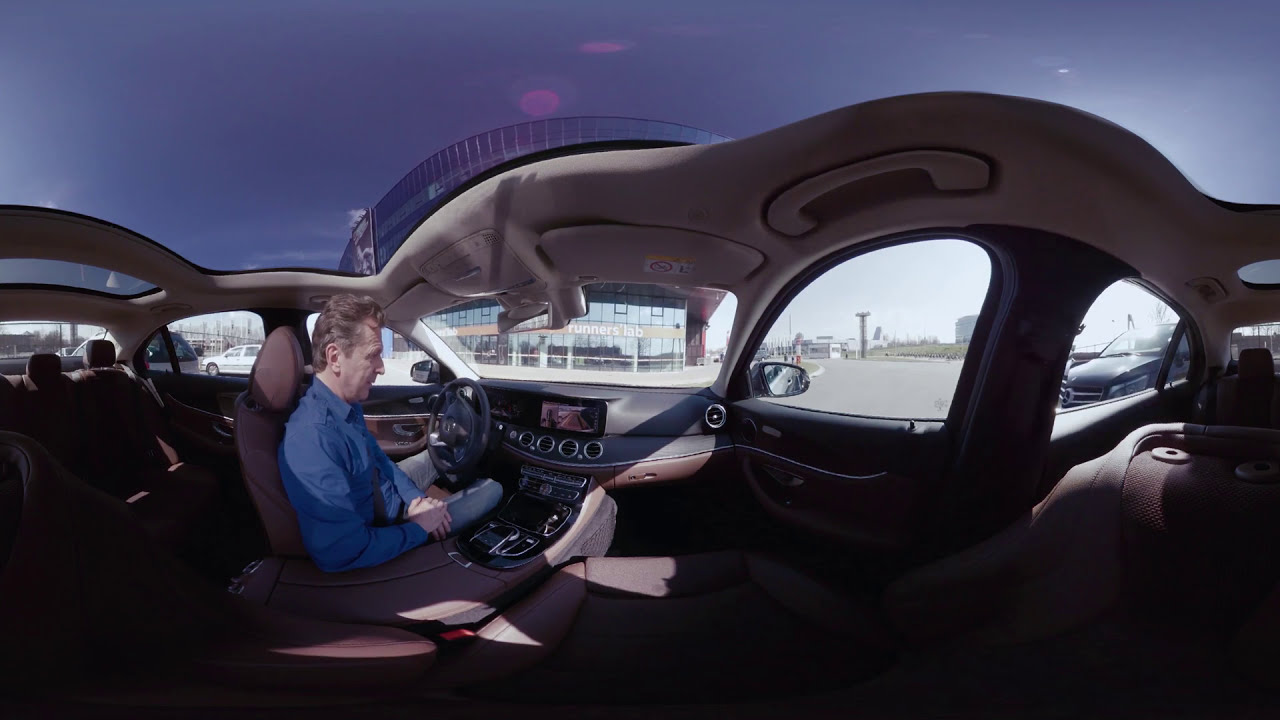The image captures the interior of a vehicle in a detailed 360-degree panorama view that has been converted into a flat format. Central to the image is an older Caucasian man, likely in his mid-40s to early 50s, with light sandy brown hair. He is seated in the driver's seat, wearing a long-sleeve blue button-up collared shirt paired with blue jeans. His hands are folded in his lap as he looks down at a control console equipped with a backup camera display. The vehicle features luxurious brown leather bucket seats, and a striking glass roof that allows a clear view of the sky above. Surrounding the driver, we can see the expansive layout: to his left, the empty back row of passenger seats; to his right, the front passenger seat and door, through which a building and other vehicles are visible. The light tan interior roof complements the scene, adding to the spacious and airy atmosphere of the car's interior.